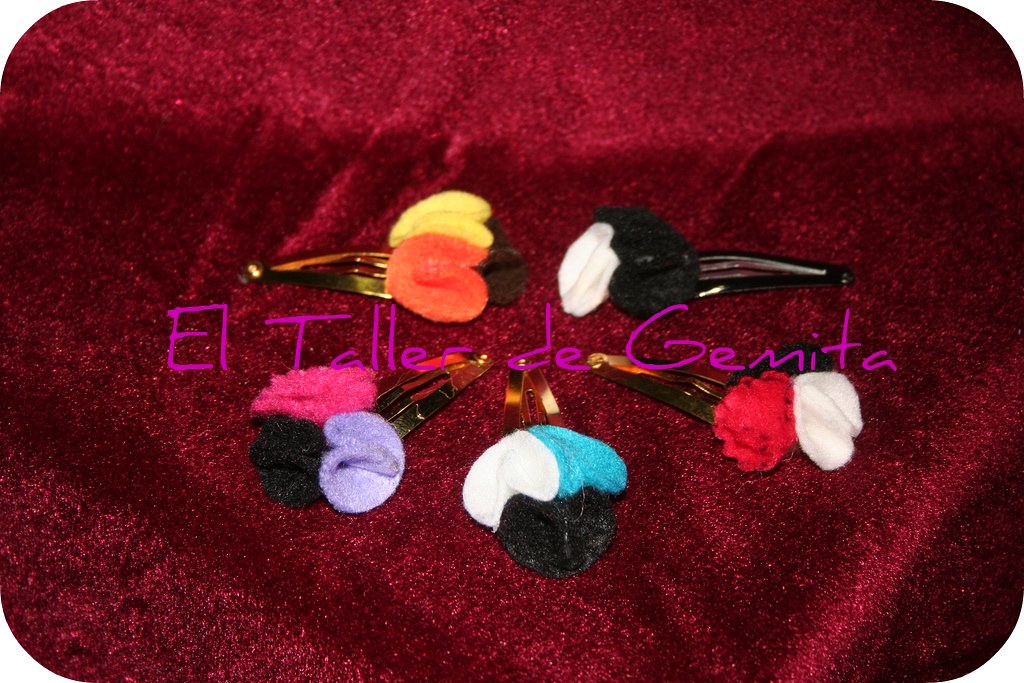The image features a deep red, almost maroon, textured background that appears to be either felt or velvet, giving it a slightly shiny finish. Prominently displayed in the center of the image is text in Spanish, reading "El Taller de Gemita" in a purple font. Below the text, there are six distinct hair clips arranged neatly. Five of these clips have a brown, bronze hue, while one is black. Each clip is adorned with small, colorful cloth puffs resembling flowers at their ends. The floral decorations come in various color combinations, including yellow, orange, and brown; black and white; pink, black, and lilac; white, blue, and black; and black, red, and white. The intricate details of the cloth puffs add a delicate, whimsical touch to the overall composition of the image.